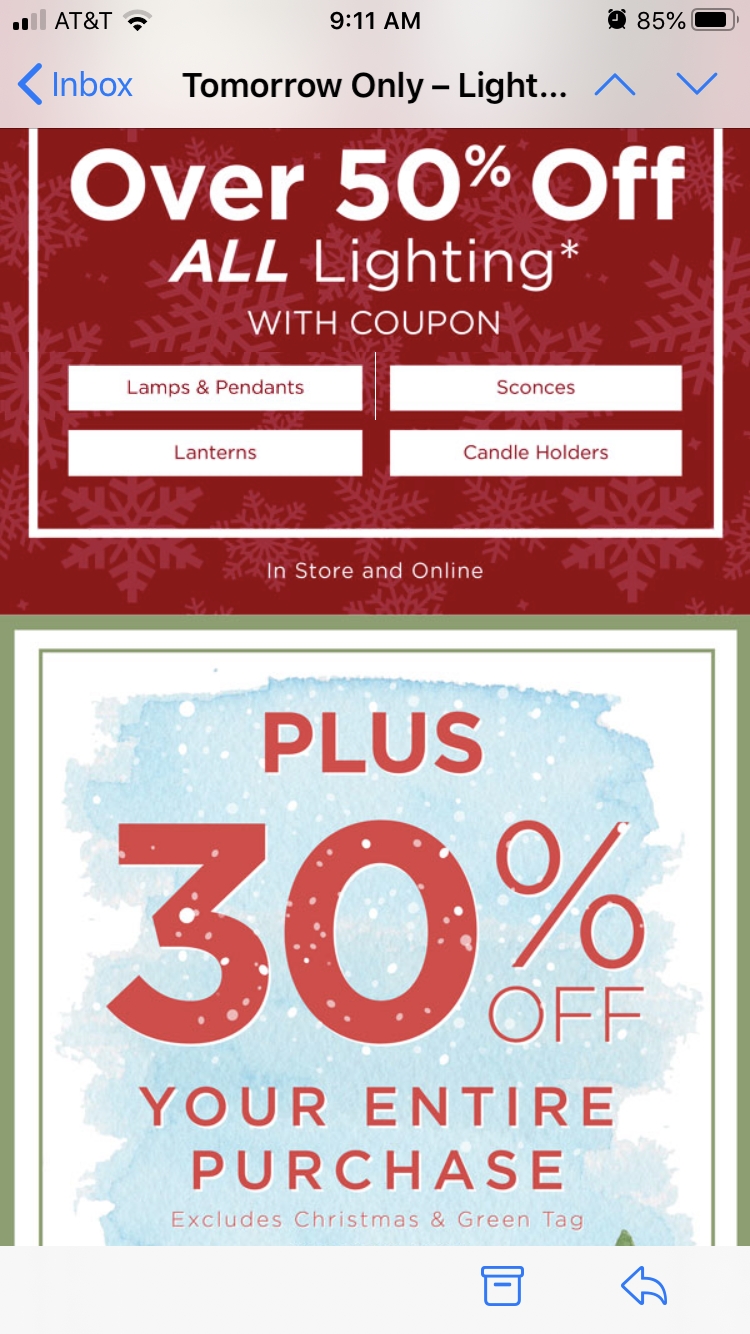The image is a vertical advertisement screenshot taken from a smartphone, likely captured from someone's email app. The top of the screen features a gray bar extending across its width, with a subtle pinkish-red light that adds dimension. In the upper left-hand corner, typical smartphone indicators are visible: a black signal bar strength icon, the AT&T carrier name, the Wi-Fi icon, the alarm clock icon, and a battery life icon showing 85%. The time is displayed centrally as 9:11 a.m. 

On the top left, there’s a blue "Inbox" label. Across the middle, in bold black text, it reads "Tomorrow only - Light..." with expandable blue arrows. Below this header, the advertisement itself begins, set against a vibrant red background adorned with white snowflakes. The primary message, written in bold white text, announces, "Over 50% off all lighting* with coupon," listing categories such as lamps, pendants, lanterns, sconces, and candle holders, applicable both in-store and online.

Further down, there's a section with a white background encased by a green border, followed by a thin line bordering in green. This segment, with a blue, snow-like design, states in red text, "Plus 30% off your entire purchase *Excludes Christmas and green tag items."